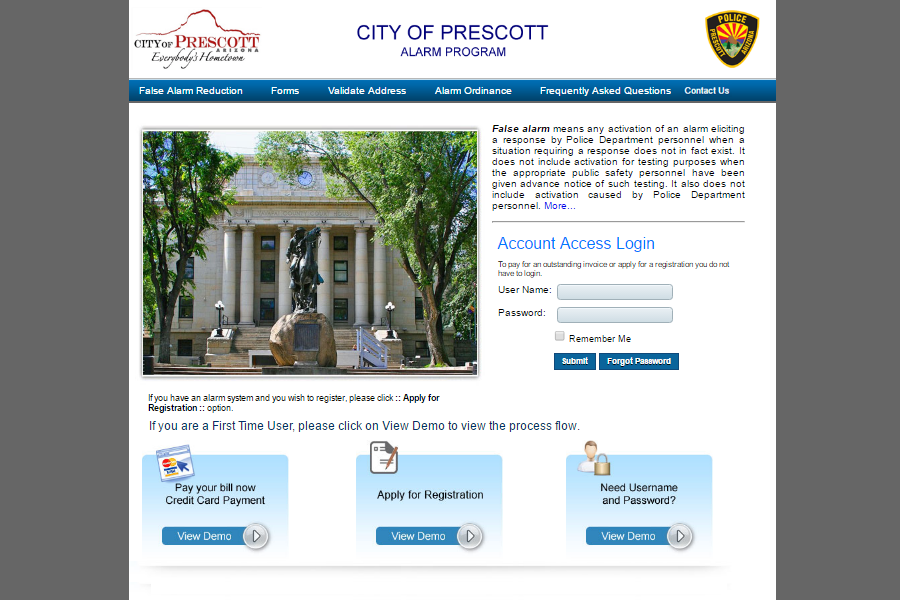The image is a landscape-oriented screenshot placed over a gray background, featuring diagonal gray stripes running from the upper left to the lower left and from the upper right to the lower right. The central focus is on the screenshot of the City of Prescott Alarm Program website.

In the upper right corner of the image, the emblem of the Prescott, Arizona Police Department is displayed. In the upper left corner, the logo for the City of Prescott, featuring the slogan "Everybody's Hometown," is visible. Known landmarks, such as Embry-Riddle Aeronautical University, are associated with this area.

The website has several tabs across the top: "False Alarm Reduction," "Forms," "Validate Address," "Alarm Ordinance," "Frequently Asked Questions," and "Contact Us." 

On the left side of the image, there is a visual depiction resembling City Hall, featuring a clock tower and a statue of a person on a horse, adding a touch of local character.

On the right side, detailed information about false alarms is provided: "A false alarm means any activation of an alarm eliciting a response by the police department personnel when a situation requiring a response does not in fact exist. This does not include activation for testing purposes when the appropriate public safety personnel have been given advance notice of such testing. It also does not include activation caused by police department personnel themselves."

Below this text, the "Account Access" section is visible, offering a form to either pay an outstanding invoice or apply for alarm registration without requiring a login. For those who need to log in, there are fields for a username and password, with an option to check "Remember Me." Two buttons are present below these fields: "Submit" and "Forgot Password."